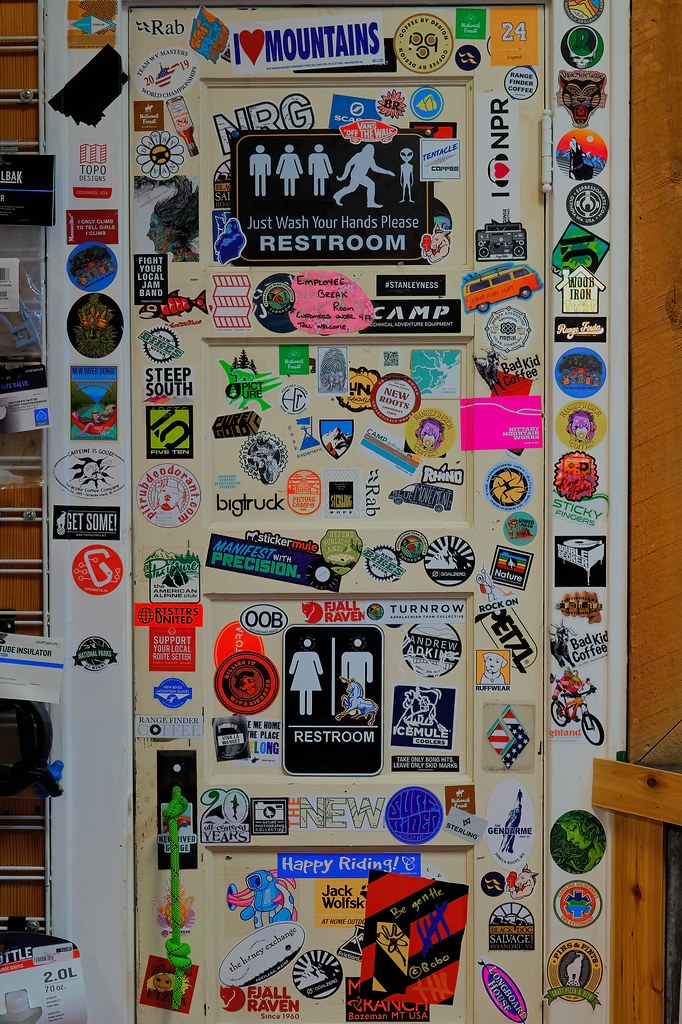The photograph is an intricate close-up of a door inside someone's home, showcasing a collection of diverse stickers. The beige door, flanked by a white frame and wooden walls, is adorned from top to bottom with a medley of colorful and eclectic stickers and signs. Central to the display is a restroom sign featuring a black background, a white border, and white silhouettes of a man and a woman, with a blue unicorn whimsically placed over the man. At the top right of the door is another black sign with an orange frame that reads "Just wash your hands, please" in white text, accompanied by illustrations of three people and a Bigfoot. Various other stickers crowd the space, proclaiming phrases like "I love mountains," "I love NPR," "bad kid," "Jack Wolf," "sky Falls," "NRG," "Ice Mule," and "Reb." The vivid colors in the collage range from hot neon pinks, bright oranges, greens, and blues to reds, whites, forest greens, blacks, grays, and burgundies. The stickers are meticulously positioned, making the door a vibrant mosaic of personal expression set against the practical setting of a bathroom entrance.